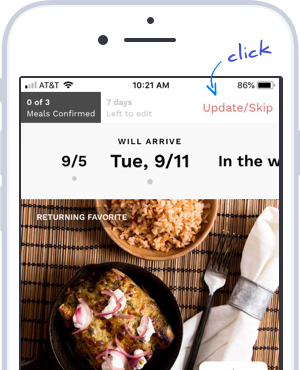**Detailed Caption:**

The image is a screenshot from a smartphone displaying details about an upcoming meal kit delivery, likely related to a meal subscription service. The phone, connected to the AT&T network, shows the current date as September 5 and the time as 10:21 a.m. The delivery is scheduled for Tuesday, September 11, with a clear image of the meal to be delivered prominently featured. Above the image, there's an option highlighted in blue allowing the user to "Update or Skip" the delivery, which suggests they can either change the delivery date, select a different meal kit, or cancel the current order. The text "Returning Favorite" indicates that this particular meal is a popular choice previously ordered by the user. Overall, this screenshot informs the user about the upcoming meal kit, providing them with options to manage their delivery before the specified date.